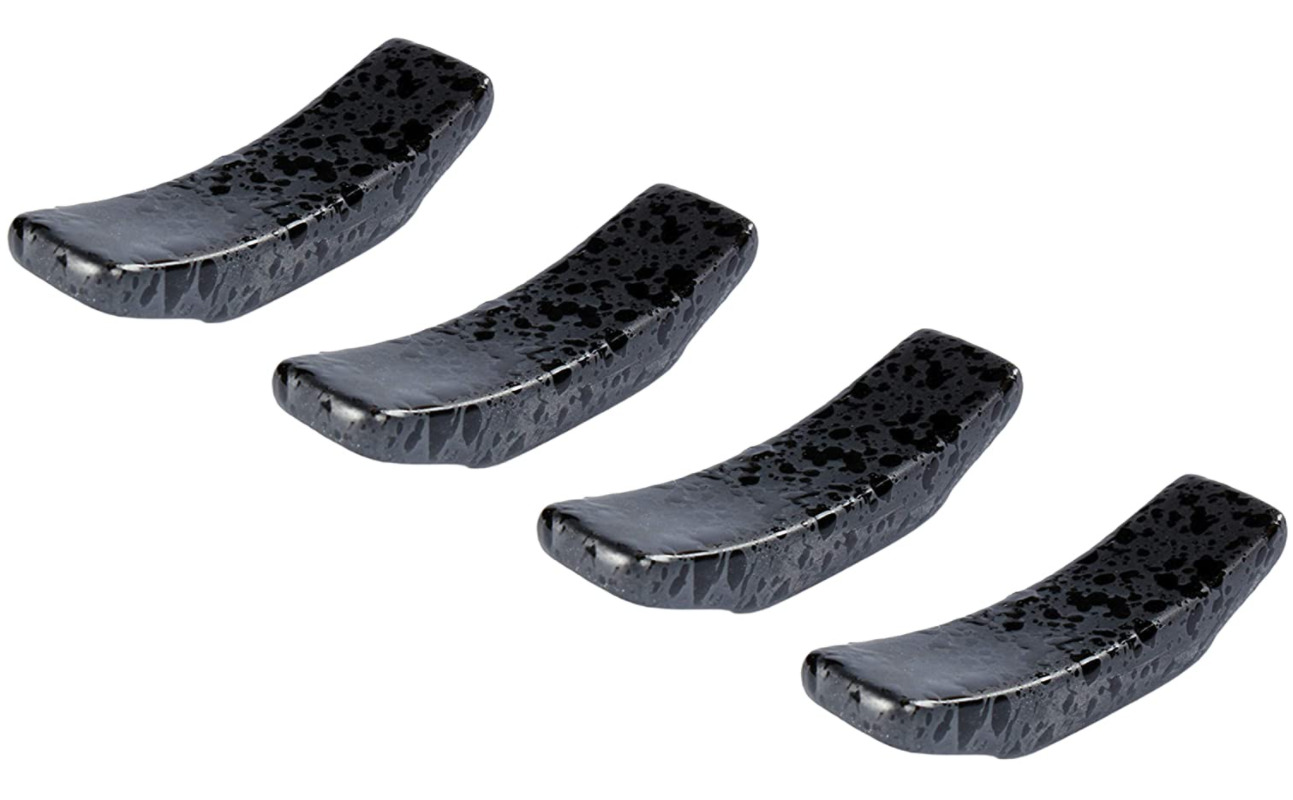The photograph captures a set of four automotive brake pads arranged diagonally from the top left to the bottom right against a stark white background. These brake pads, primarily gray with black bases, are shaped like inverted U's, reflecting the gentle curve designed to interface with the brake tread for optimal performance. The pads also feature shiny spots that catch the light from the camera, highlighting their metallic or stone-like texture. The overall image is sharp and well-lit, emphasizing the details and symmetrical arrangement of the pads, with no additional objects, text, or people present in the frame.